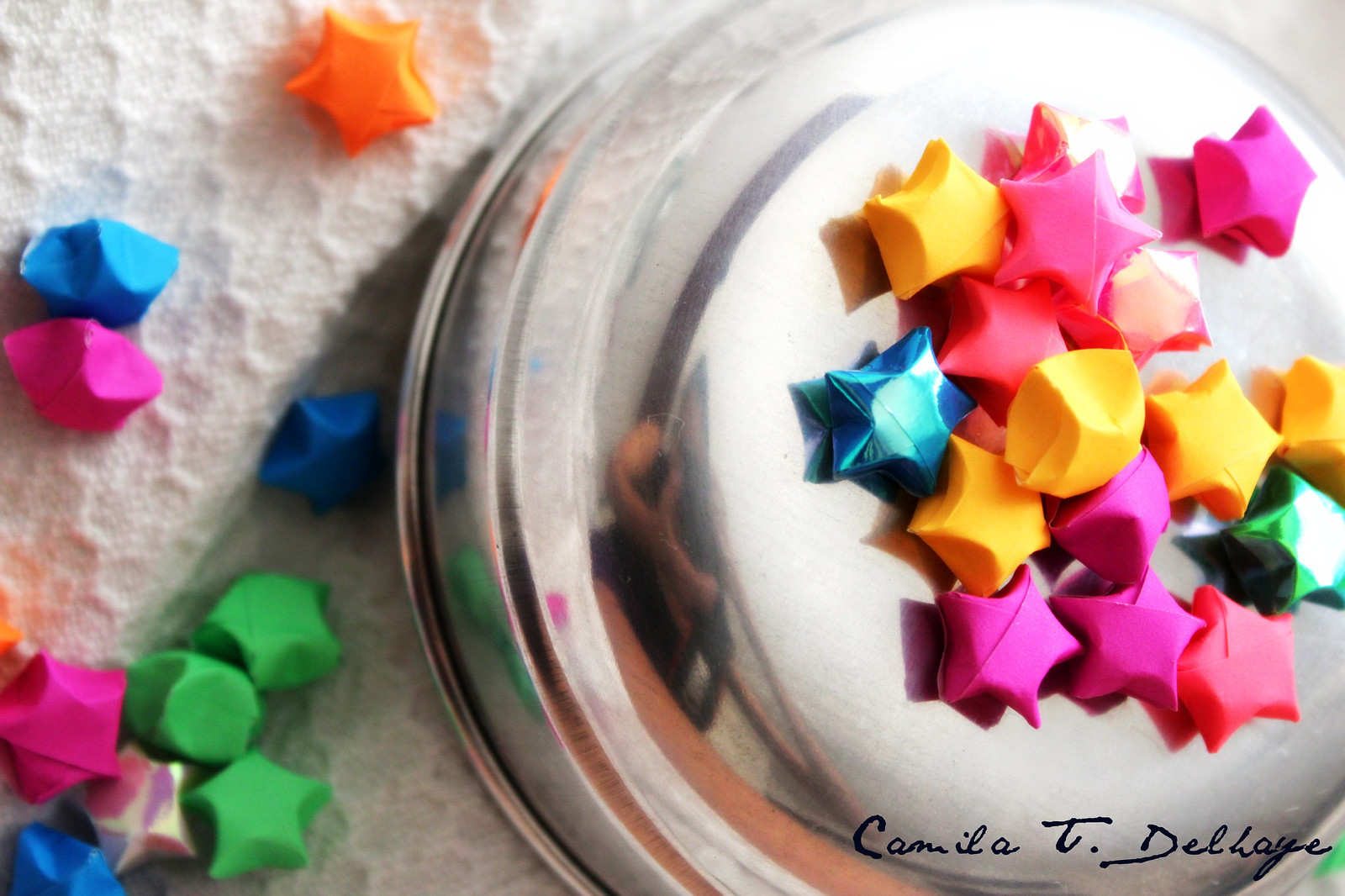The photograph features an overturned stainless steel bowl, approximately the size of a cereal bowl, positioned against a white background with a honeycomb-like texture, which could be a knitted blanket or tablecloth. Scattered both on top of the bowl and to its left are numerous small, colorful star-shaped beads or folded paper stars in metallic blue, green, yellow, pink, silver, and orange hues. In the bottom right corner, the image is signed "Camilla T. Delhay" in cursive, although the exact spelling is somewhat difficult to decipher.